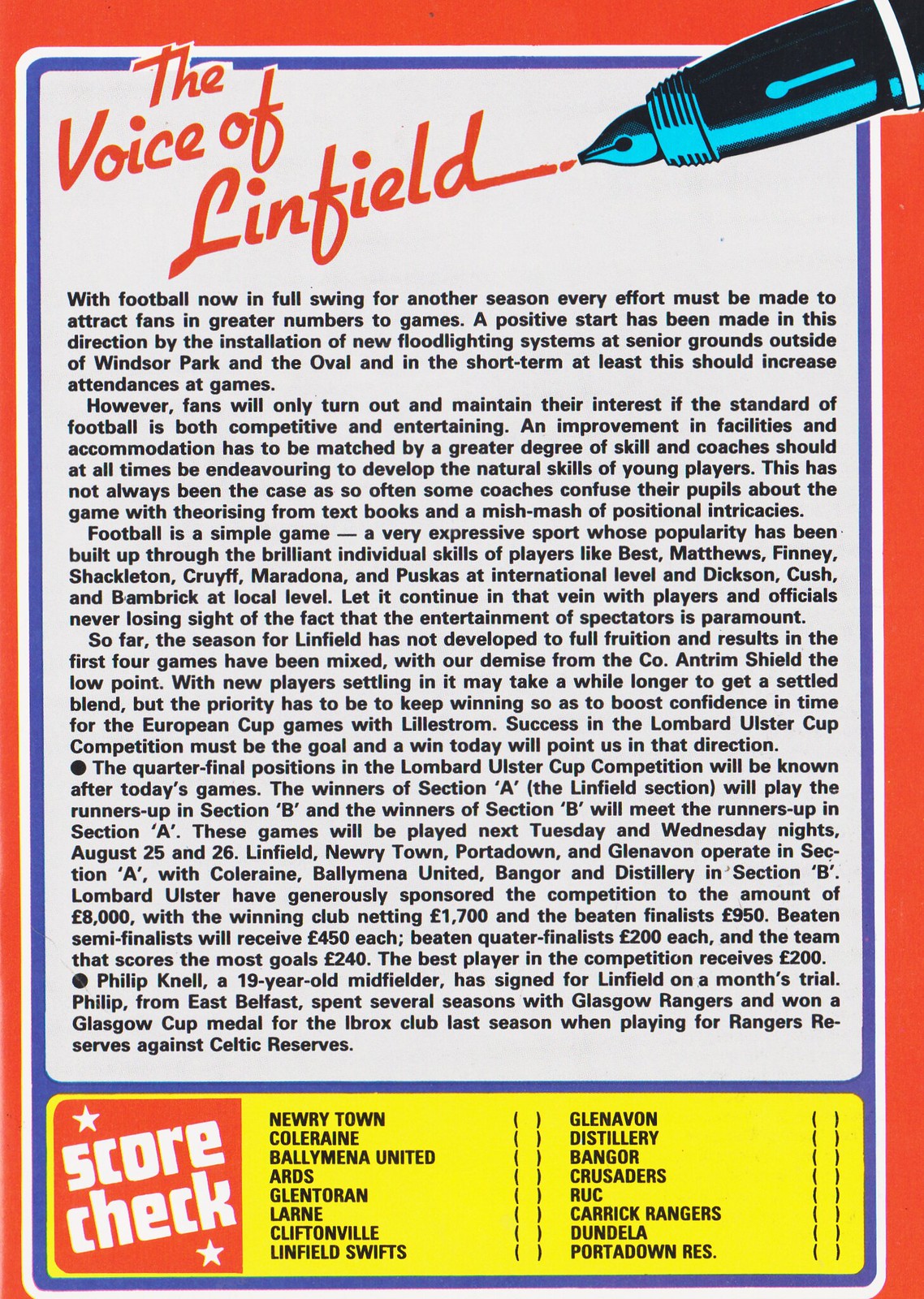This color image from a vintage magazine, titled "The Voice of Linfield," features a detailed layout with a distinctive red background and border, which encases a thin blue inner border. Inside this frame rests a white background that hosts the main content. In the top corner, an old-fashioned ink pen is illustrated diagonally, as if it has just finished writing the article's title in elegant script.

The headline reads "The Voice of Linfield," placed prominently at the top. Below, the article discusses the current football season, emphasizing the need to attract more fans to games. It highlights the recent installation of new floodlighting systems at senior football grounds outside of Windsor Park and the Oval, which aims to boost attendance in the short term. The text argues that fans' continued interest depends on the competitive and entertaining quality of the football played. It criticizes some coaches for confusing players with over-complicated theories and stresses the importance of nurturing natural skills, citing legendary players both internationally and locally.

The article also reviews Linfield's mixed results in the early season, mentioning the team's exit from the CO Antrim Shield as a low point. It suggests that new players need time to gel, but underlines the importance of maintaining wins to build confidence, especially for upcoming European Cup games against Lillestrom. The piece concludes with a note on the significance of success in the Lombard Ulster Cup competition.

Towards the bottom, there is a "Scorecheck" section featuring various teams such as Newrytown, Colerain, Ballymena United, and others, set within a yellow box. This section is accompanied by a red square highlighting scores with white text. The entire page is framed with blue and red trimming, adding to the vintage aesthetic of the magazine layout.